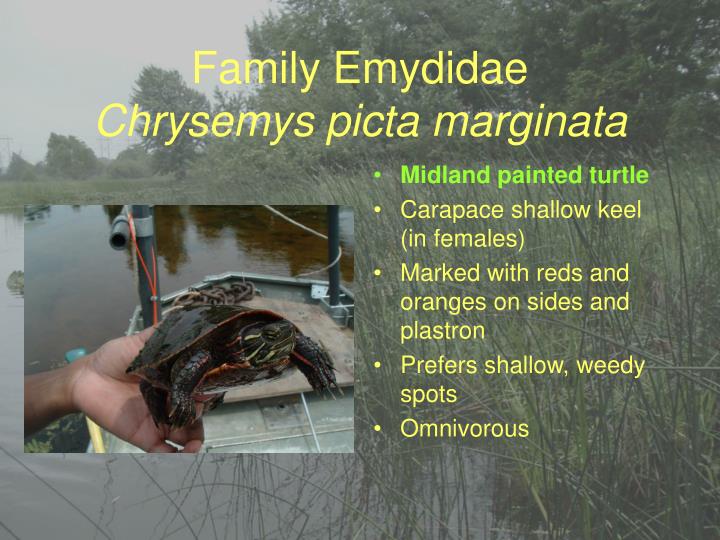The infographic features a detailed educational slide about the Midland Painted Turtle, known scientifically as Chrysemis picta marginata from the family Emydidae. At the center of the slide, a vibrant photograph captures a person holding a medium-sized, hand-sized turtle up to the camera. This turtle has a distinct black shell with striking red rims around the edges, black legs, and a head adorned with yellowish green stripes.

The background of the slide presents a serene, slightly washed-out marshland scene with tall green reeds and scattered trees set against a grayish sky, likely allowing the text to be more legible. A boat or dock is visible behind the main photograph, indicating the turtle's natural habitat.

At the top of the slide, yellow text identifies the scientific classification, "Family: Emydidae, Chrysemis picta marginata." Below the photo, five bullet points explain key characteristics of the Midland Painted Turtle:
1. **Midland Painted Turtle**
2. **Carapace with a shallow keel in females**
3. **Marked with reds and oranges on sides and plastron**
4. **Prefers shallow, weedy spots**
5. **Omnivorous**

Overall, the slide blends informative text with a captivating image to provide a comprehensive overview of the Midland Painted Turtle, set against an evocative natural backdrop.